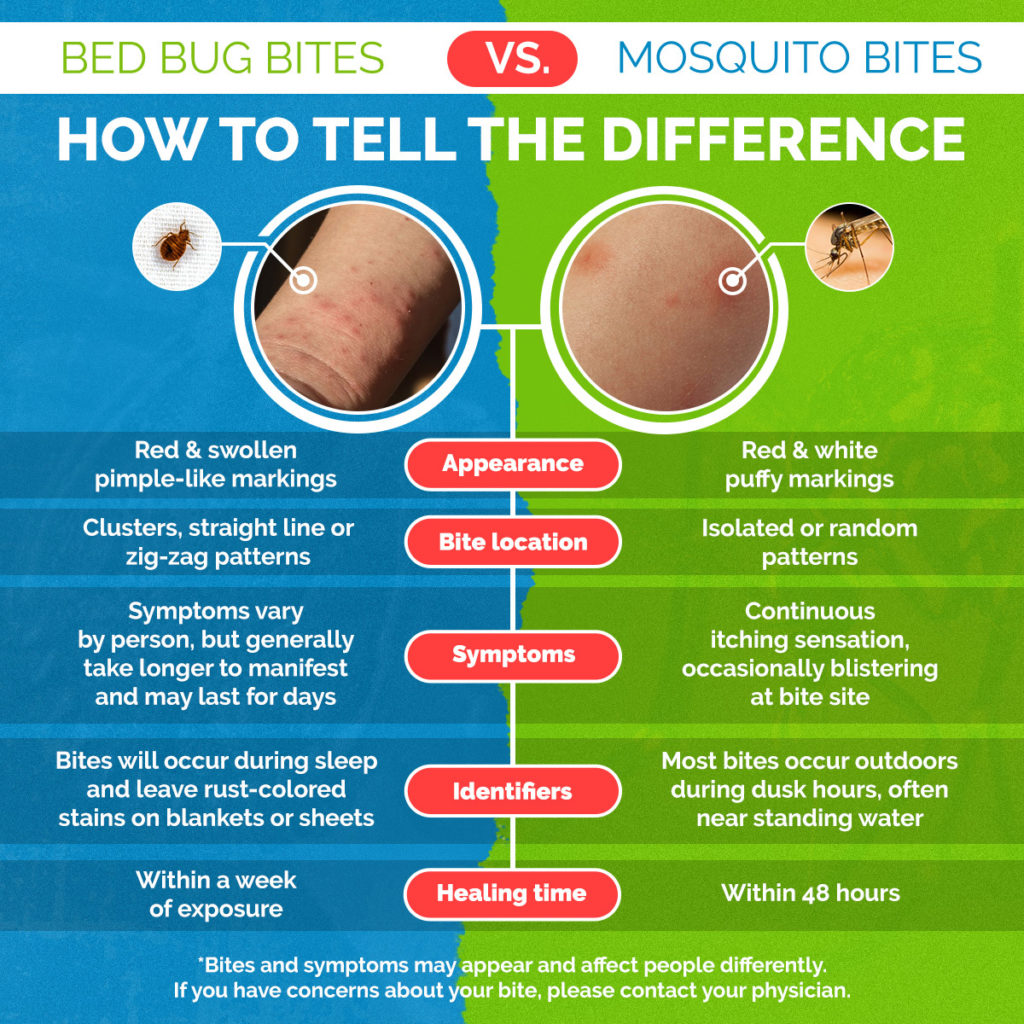This detailed infographic, titled "Bed Bug Bites vs Mosquito Bites: How to Tell the Difference," is divided into two distinct sections: a blue left side for bed bug bites and a green right side for mosquito bites. At the top, the large title is clearly visible in white font. The infographic features two large circles; the left circle depicts a human hand with bed bug bites, and the right circle showcases an area of skin with mosquito bites.

Accompanying each of these circles are smaller circles illustrating the respective insect— a tick-like bed bug on the left and a mosquito on the right. The diagram is divided into five categories, each marked by red horizontal buttons in the center: Appearance, Bite Location, Symptoms, Identifiers, and Healing Time. Detailed information under each category helps differentiate bed bug bites from mosquito bites.

For bed bug bites, the infographic notes that the appearance includes red, swollen, pimple-like markings, often in clusters, straight lines, or zigzag patterns. Conversely, mosquito bites are described as red and white puffy marks, typically appearing in isolated or random patterns. Under each category, additional symptoms and identifiers are listed alongside healing time estimates.

At the bottom of the infographic, a disclaimer advises that bites and symptoms may vary among individuals and recommends contacting a physician if concerns arise. The entire infographic is visually unified with a medical theme and well-organized details, making it an informative guide for distinguishing between bed bug and mosquito bites.